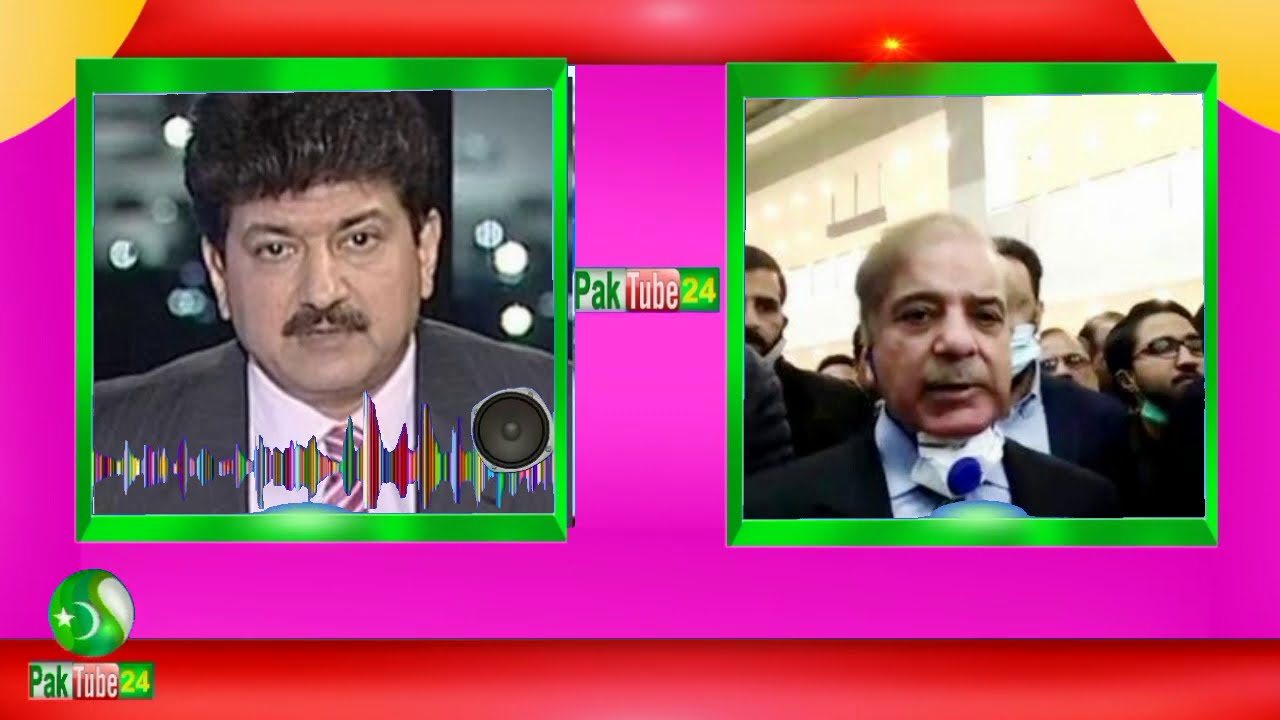This is a wide rectangular digital image, seemingly a screenshot of a TV or YouTube channel, featuring a vibrant and structured layout. The background is predominantly red, accented by curved white shapes in the top left and right corners, resembling suns. A large pink rectangle spans the center of the image, bordered by a mix of red and yellow corners, providing a backdrop for two prominently displayed screens.

The two screens are enclosed within neon bright green gradient frames. On the left screen, there is a man wearing a gray suit jacket, a white collared shirt, and a purple tie with white stripes. He sports a dark mustache and thick brown hair, reminiscent of a 60s image. On the right screen, another man also wearing a suit appears, with a mask positioned around his neck. He has light brown, thinning hair and a mustache. The screens suggest a dynamic between a studio broadcaster and a field correspondent.

Positioned between the two screens, the channel name "PacTube 24" is clearly visible. The word "PacTube" is divided into segments with "PAC" in green letters on a white background, "tube" in white letters on a red background, and "24" in yellow letters on a green background. This logo can also be seen in the bottom left corner of the image. Together, the detailed elements and vibrant colors suggest a lively and engaging broadcast.